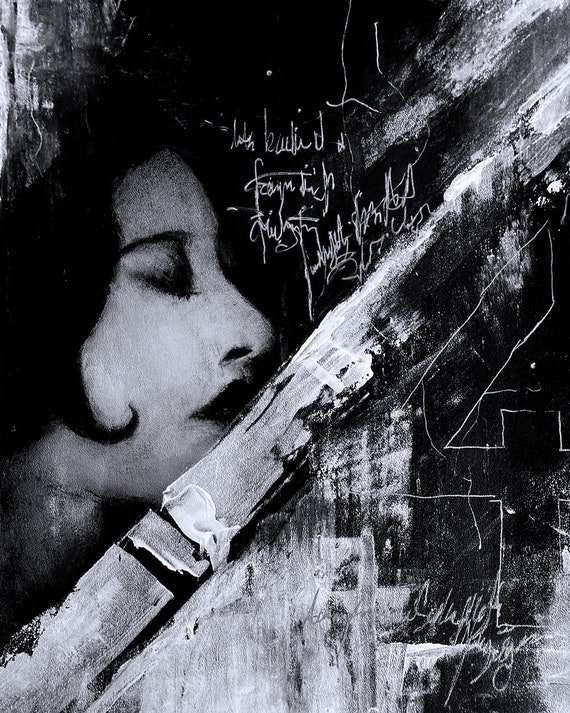This black and white artistic drawing features a striking woman's face in profile on the left-hand side, her eyes closed and her expression serene. The background is a deep black, seamlessly blending with her dark hair that curls forward around her cheek, creating a contrast against her very white, light face. Her thin eyebrows, dark eyeshadow, and bold black lipstick add to her dramatic appearance. Distressed white paint and gray elements interplay with the black background, creating an abstract, textured effect. Strokes from a chisel-like tool scrape across the canvas, adding to the distressed feel. Illegible scribbled writing, possibly containing the word "beautiful," is scattered throughout the image, enhancing the abstract theme. The overall composition is evocative and mysterious, with each element blending into a cohesive and compelling visual narrative.